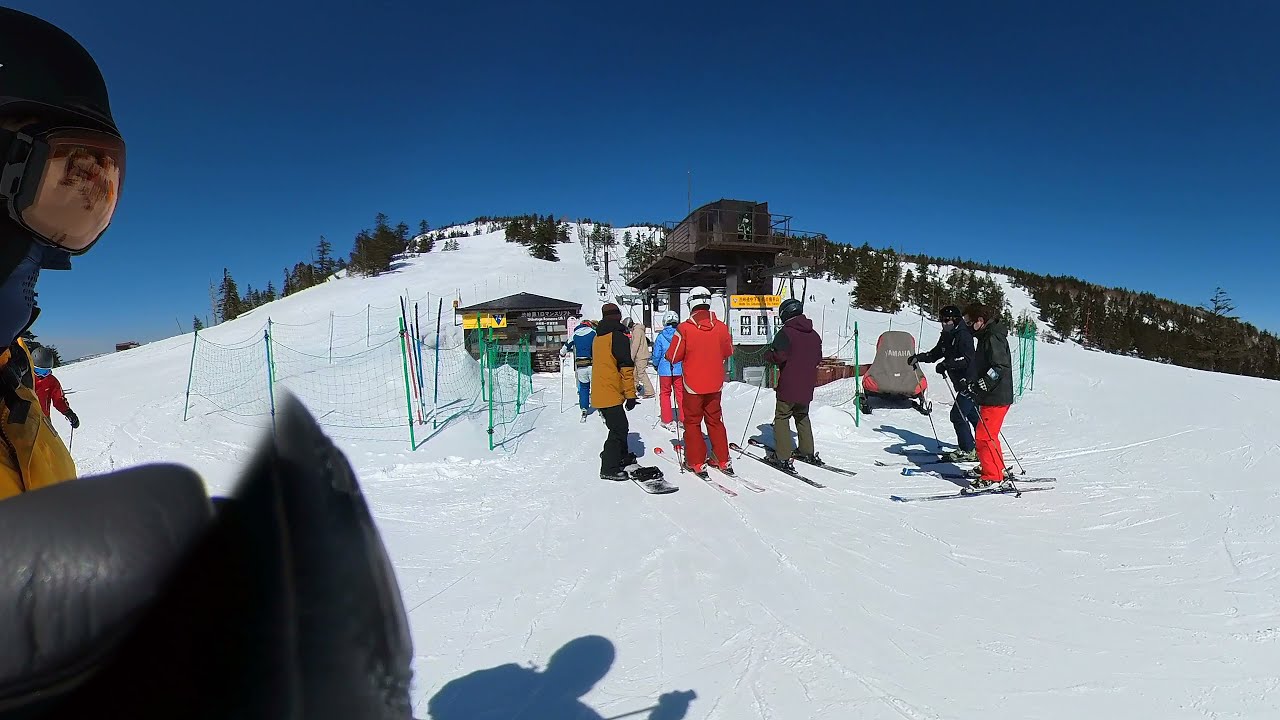In this detailed photographic image taken outdoors on a clear day, a group of skiers and one snowboarder are captured at the base of a snow-covered mountain. They are queued up to board a ski lift, their backs turned to the camera. The scene is bustling with action as the skiers, dressed in colorful, insulated winter wear, prepare for their ascent.

From left to right, we see a person in a blue jacket paired with dark blue pants and a helmet of matching colors. Next, there is an individual in a brown jacket and gray pants, wearing a gray helmet. Moving right, a skier stands in a bright red jacket and red pants with a white helmet. Next to him, there is another skier in a blue jacket and red pants. In front of this person, we notice a man wearing a brown and black jacket standing by his snowboard. Further to the right, another skier is visible in a black jacket, red pants, and a helmet, alongside another individual dressed in all black with a helmet. 

In the background, there are buildings associated with the ski lift, one of which has a gabled roof. Although there is text on the signage, it is too small to be legible. The blue sky and snow-laden mountain top with scattered evergreen trees provide a picturesque backdrop. The snow is marked with numerous ski streaks, evidence of the well-traveled slope. A shadow of a person is cast on the snow to the left, and what appears to be an arm with a red marking is also visible on the far left. The scene encapsulates the lively and dynamic nature of a ski day on the mountain.